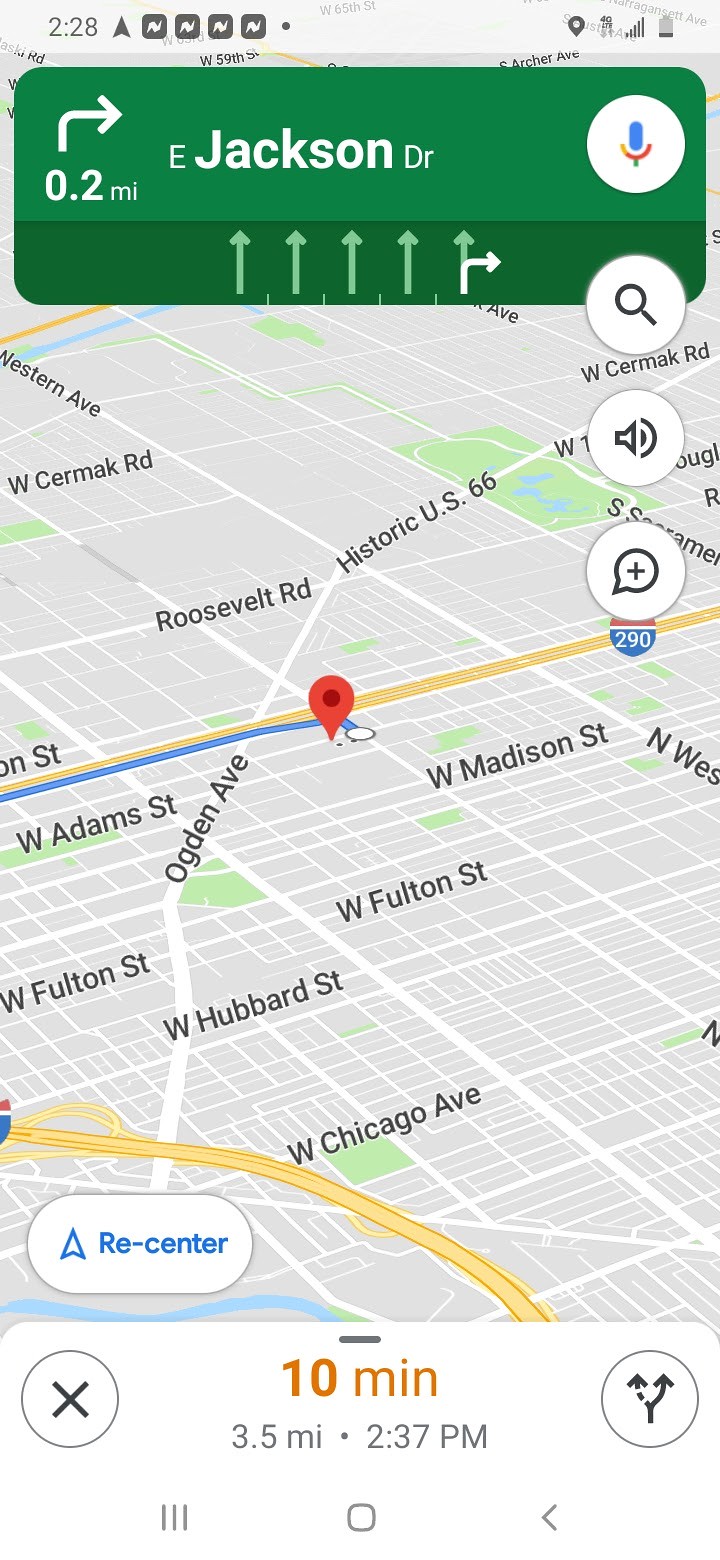The image shows a screenshot from a mapping app displaying directions in progress. At the top of the image, within a green rectangle, is a navigation instruction indicating a turn in 0.2 miles. The instruction to "Turn right onto East Jackson Drive" is displayed in bold white text alongside a right-turn arrow. To the right of this rectangle is a cylindrical white button featuring a microphone icon. Below this main button are three smaller cylindrical white buttons: one with a magnifying glass icon, another with a speaker icon, and a third with a chat bubble and a plus sign.

The main portion of the image features a diagonal bird's-eye view of various streets. A blue line traces the route to the final destination, pinpointed by a red balloon icon. At the bottom of the image, a white rectangle provides additional trip details: in orange text, it notes a 10-minute travel time over 3.5 miles, with an estimated arrival time of 2:37 PM in smaller gray text. To the left of this information box is a circular button with a gray border displaying an 'X', likely for canceling or closing the directions. On the right side, a similar button shows a splitting path arrow symbol, which could indicate a rerouting option.